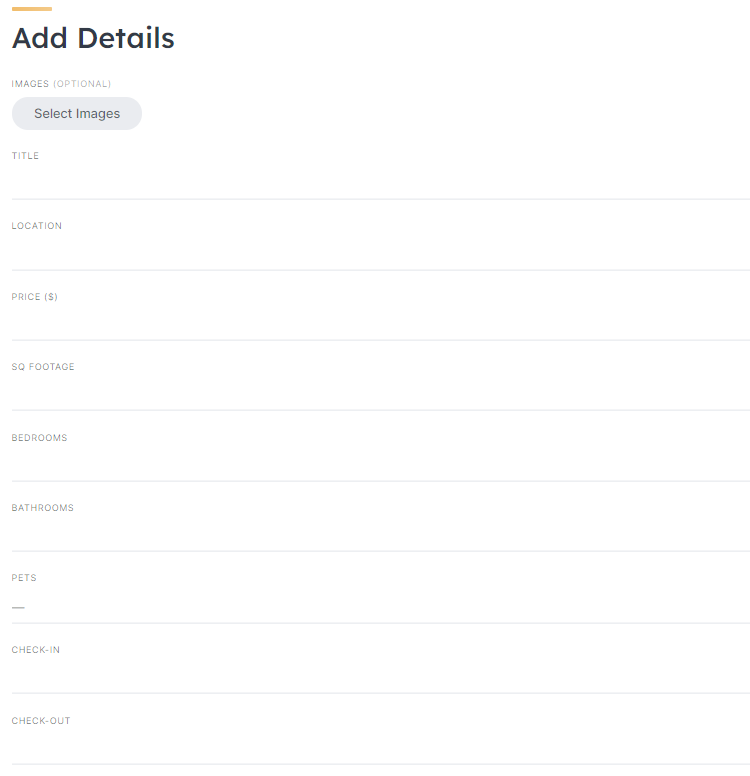This image displays a detailed form designed for users to add extensive information about a property, likely for short-term rentals similar to Airbnb. At the very top, there is a field labeled "Add Details," followed by an optional section for uploading images with a corresponding "Select Images" button, allowing users to upload photos from their PC or phone. Below this, several fields are arranged for inputting various property details. These fields include: Title, Location, Price in dollars, Square Footage (SQ footage), Bedrooms, Bathrooms, Pets, Check-in, and Check-out times. This comprehensive form provides ample space in each field for users to input detailed and relevant information about their property, ensuring a thorough listing.